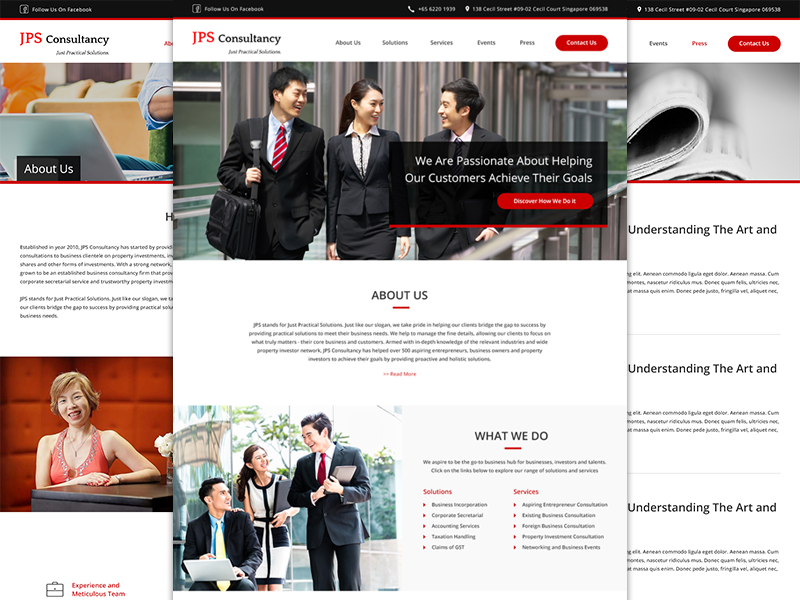A detailed caption for the given image could be:

"A screenshot depicting a layered view of three overlapping pages from the JPS Consultancy website. The JPS Consultancy logo is prominently displayed at the top left corner, with 'JPS' in red and the rest of the text in black. Spanning the top of the page is a sleek white menu bar featuring six links: 'About Us,' 'Solutions,' 'Services,' 'Events,' 'Press,' and a pill-shaped 'Contact Us' button. Dominating the header is a banner image of three professionals of Asian descent dressed in business attire. In the center is a woman, flanked by two men, one of whom is holding a laptop bag."